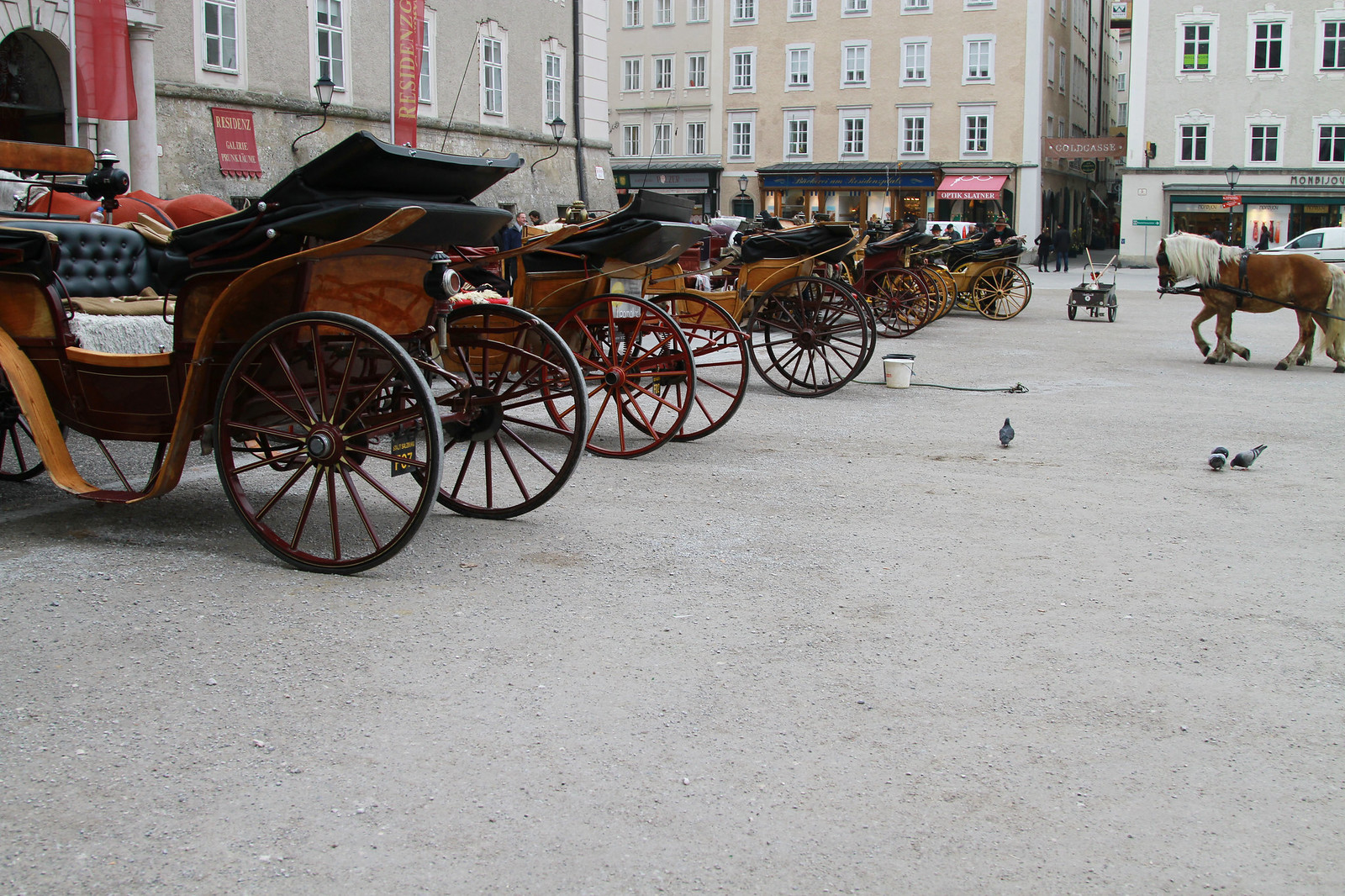The photograph depicts a row of approximately a dozen horse-drawn carriages, each equipped with collapsible canopies pulled back in the down position, parked closely side by side on a concrete surface. This setting is situated within a European square characterized by diverse architectural styles, including buildings with store fronts on the lower levels and apartments or houses above. The buildings exhibit muted color palettes, predominantly gray, but also feature touches of mauve from hanging banners and a pale yellow building in the background. The square includes a large courtyard populated by pigeons, adding to the daily activity of the scene. To the right, a brown horse, adorned with a saddle and black harness, mane flowing over its face, is seen walking towards the carriages, suggesting it is likely another carriage horse. The overall atmosphere of the photo suggests it was taken on an overcast, somewhat dreary day, likely contributing to the overall muted lighting and the impression of a tranquil, yet lively urban square.